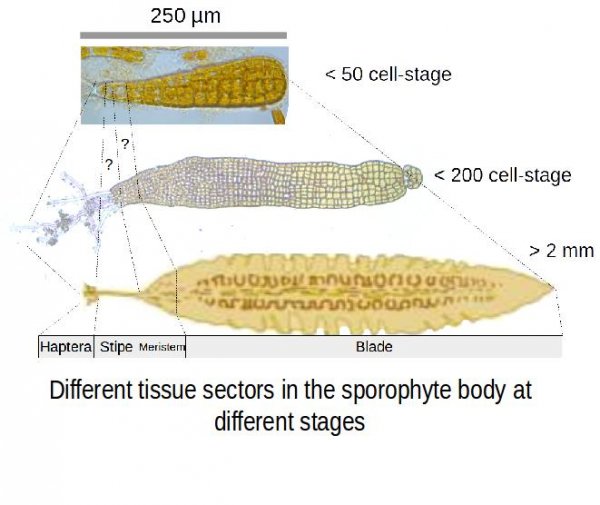The horizontal image, set against a plain white background with no visible borders, is approximately four inches high by four inches wide. At the bottom of the image, there are two rows of large black text that reads, "different tissue sectors in the sporophyte body at different stages." Above this, a horizontal thin black line is depicted with a slightly wider light gray line beneath it. The gray line contains black print that labels different tissue sectors: on the left side, "haptera," "stipe," "meristem," and on the right side, "blade."

Higher up, the image showcases three different stages of sporophyte tissue development, represented by distinct cross-sections. The first cross-section at the top is labeled "less than 50 cell stage" and appears as an oblong object with a blue outline, somewhat resembling a fish. The middle cross-section, labeled "less than 200 cell stage," features a two-toned object in light purple on the left and yellow on the right, looking like an irregularly shaped ear of corn. The third cross-section at the bottom is labeled "less than two millimeters" and resembles a feather with a light tannish-yellow color.

The caption integrates the repeated elements to highlight the image's purpose in illustrating the structural changes of sporophyte tissue at various stages, using colorful and identifiable shapes to showcase these scientific observations.